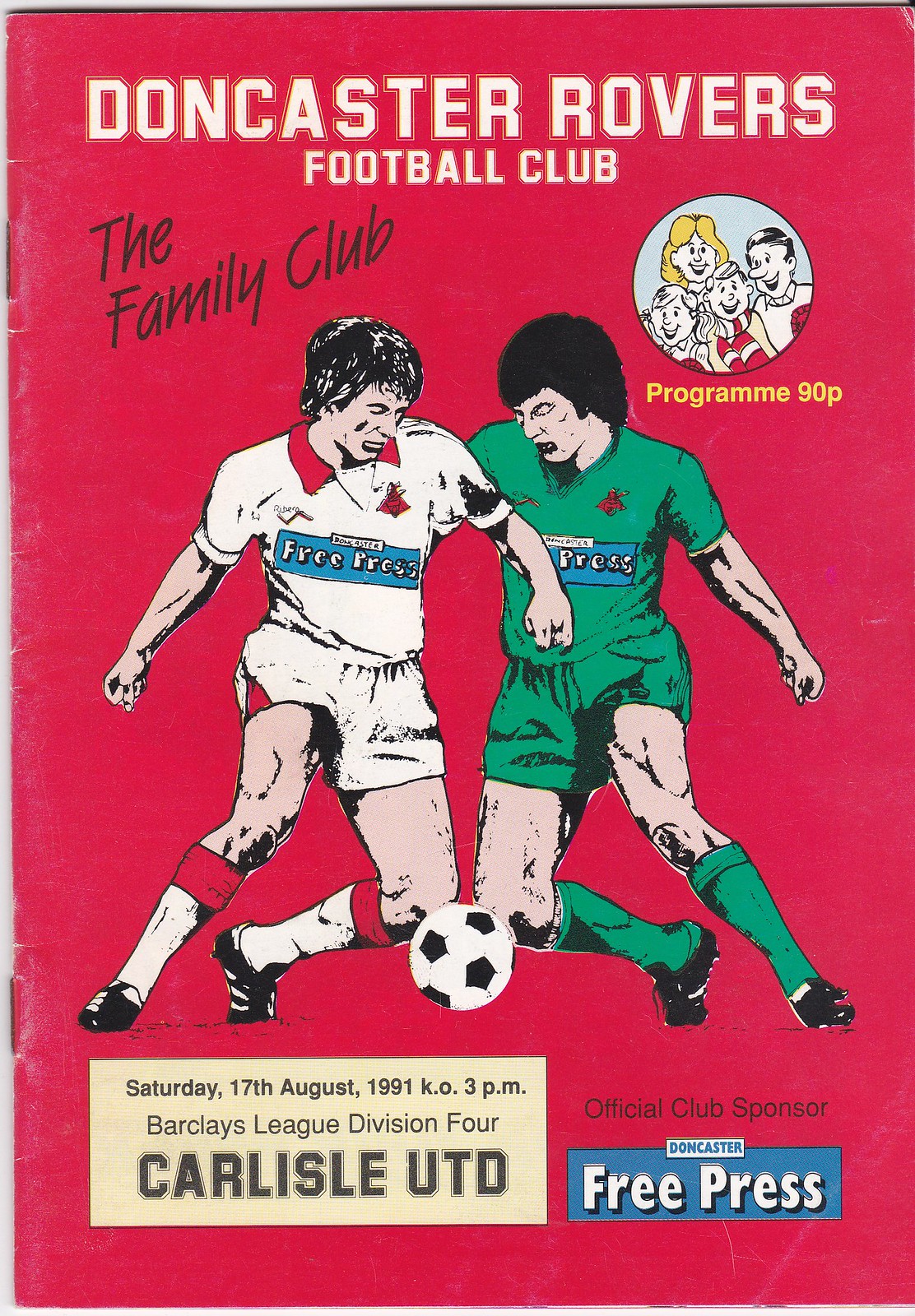The poster is a tall rectangular image designed as a front page for a sports program or pamphlet, prominently featuring the Doncaster Rovers Football Club. The top of the poster displays the bold geometric white text "Doncaster Rovers Football Club" with a thin white border. Adjacent to this text, there's a small circular drawing of a smiling family in a blue background. Below the family image, "The Family Club" is written in black handwritten letters. The pricing information "Program 90p" is positioned underneath the family.

Dominating the center of the poster, there is a vibrant depiction of two soccer players in action. The player on the left, who has light skin and is wearing a white uniform with red borders, is engaging with the ball against a player on the right, who has slightly darker skin, black hair, and a green and blue uniform. Their movements are dynamic, captured with the ball near their knees. A blue rectangle next to each player reads "Free Press."

The background of the poster is a solid pink color. Below the central image of the players, there is additional black and white text detailing event information: "Saturday 17th August 1991 KO3PM Barclays League Division 4 Carlisle UTD," and "Official Club Sponsor Doncaster Free Press," located towards the bottom right of the poster.